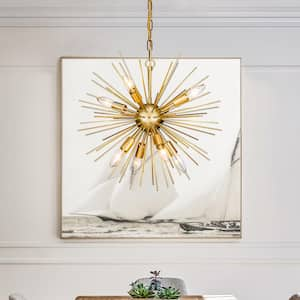The image captures a chic dining room setting with a striking centerpiece. Framed against a pristine white wall is a large, black-and-white photograph depicting two sailboats racing closely together, evoking a sense of dynamic motion and competition. In the foreground, partially obscuring this nautical artwork, hangs an elaborate chandelier. The chandelier, resembling a radiant sunburst, features numerous spikes extending outward, some adorned with light bulbs at their ends. This artistic lighting fixture hangs above a dining table, adding an intriguing, modern contrast to the classic elegance of the sailboat photograph behind it.